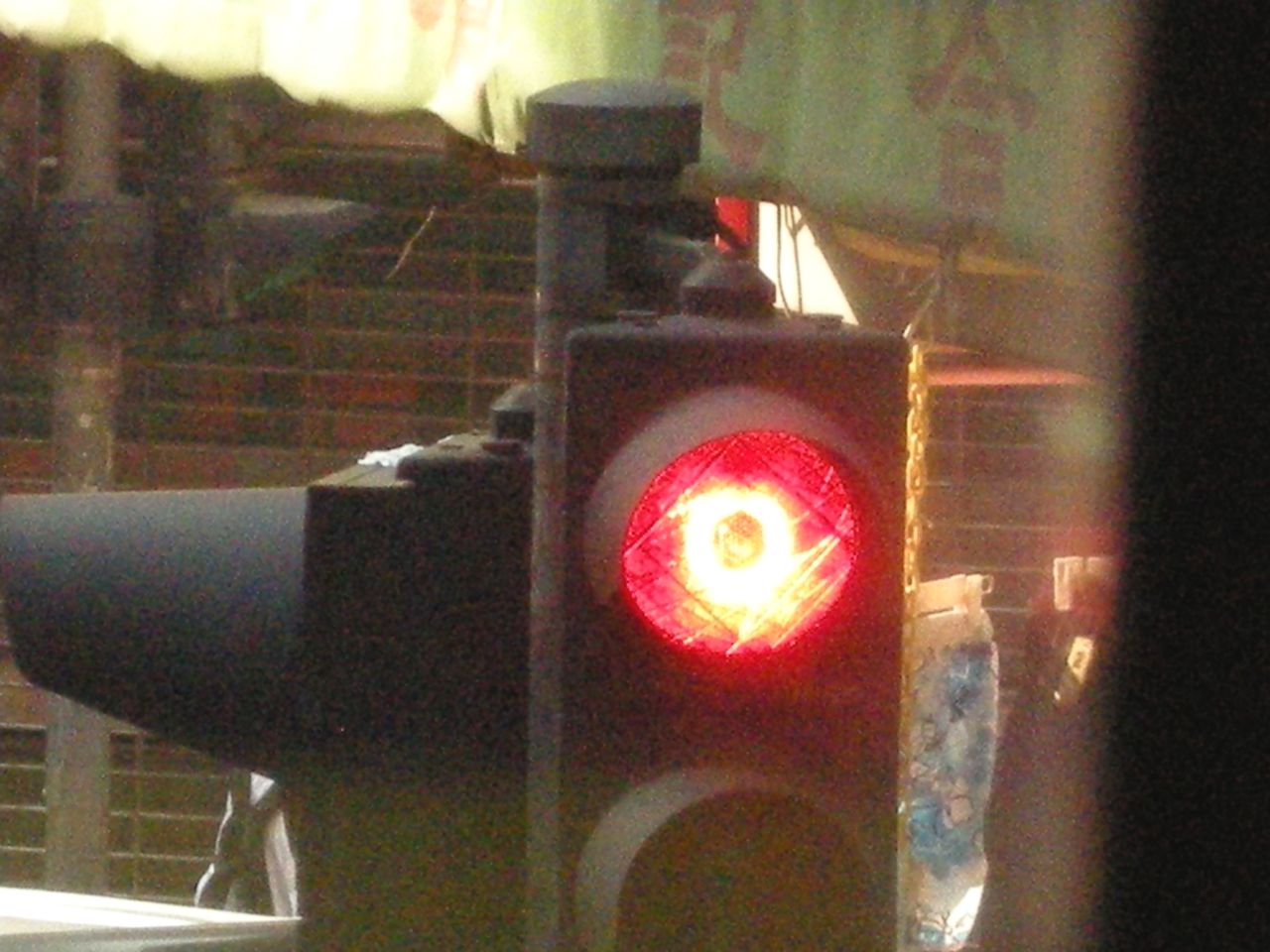A grainy close-up photograph of the top section of a traffic light, captured with a telephoto lens. The central focus of the image is the bright red glowing stop signal, which features small lines traversing its textured surface. The innermost part of the light is overexposed, creating a sun-like yellow effect. The backdrop hints at an urban setting, with a brick wall and a flag or curtain adorned with Asian symbols visible behind the traffic light. A thin black strip runs vertically down the right edge of the photograph, potentially caused by an obstruction from within the building where the shot was taken.